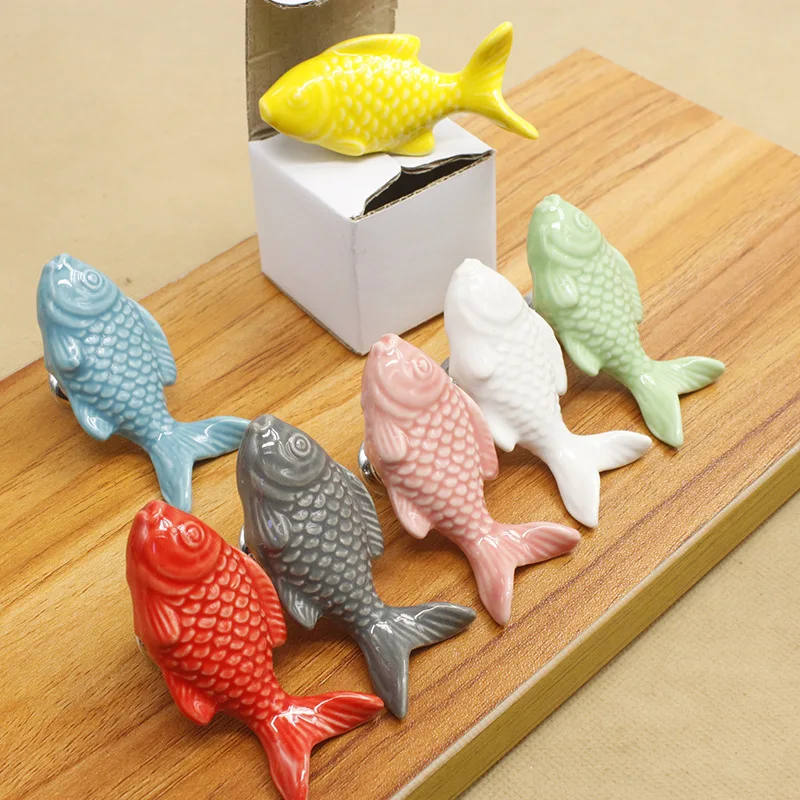In the image, a collection of ceramic fish figurines, each meticulously painted in various colors, is displayed. The cream-colored floor provides a neutral background, enhancing the vibrancy of the wooden platform upon which they rest. This wooden surface, polished to a high gloss, features a light brown grain finish and could be mistaken for a finely crafted wooden bench. At the center of this arrangement is a white, cube-shaped carton box, partially opened. Perched atop this box is a shiny yellow ceramic fish. Arrayed around the box, directly on the wooden surface, are six more ceramic fish, each adorned in a distinct hue: light blue, red, gray, pink, white, and light green. The figurines resemble goldfish or koi, displaying detailed scales, fins, and carved eyes, each with a characteristically open mouth. The meticulous arrangement and vivid colors of the ceramic fishes create a visually striking and harmonious display, blending art with simplicity.